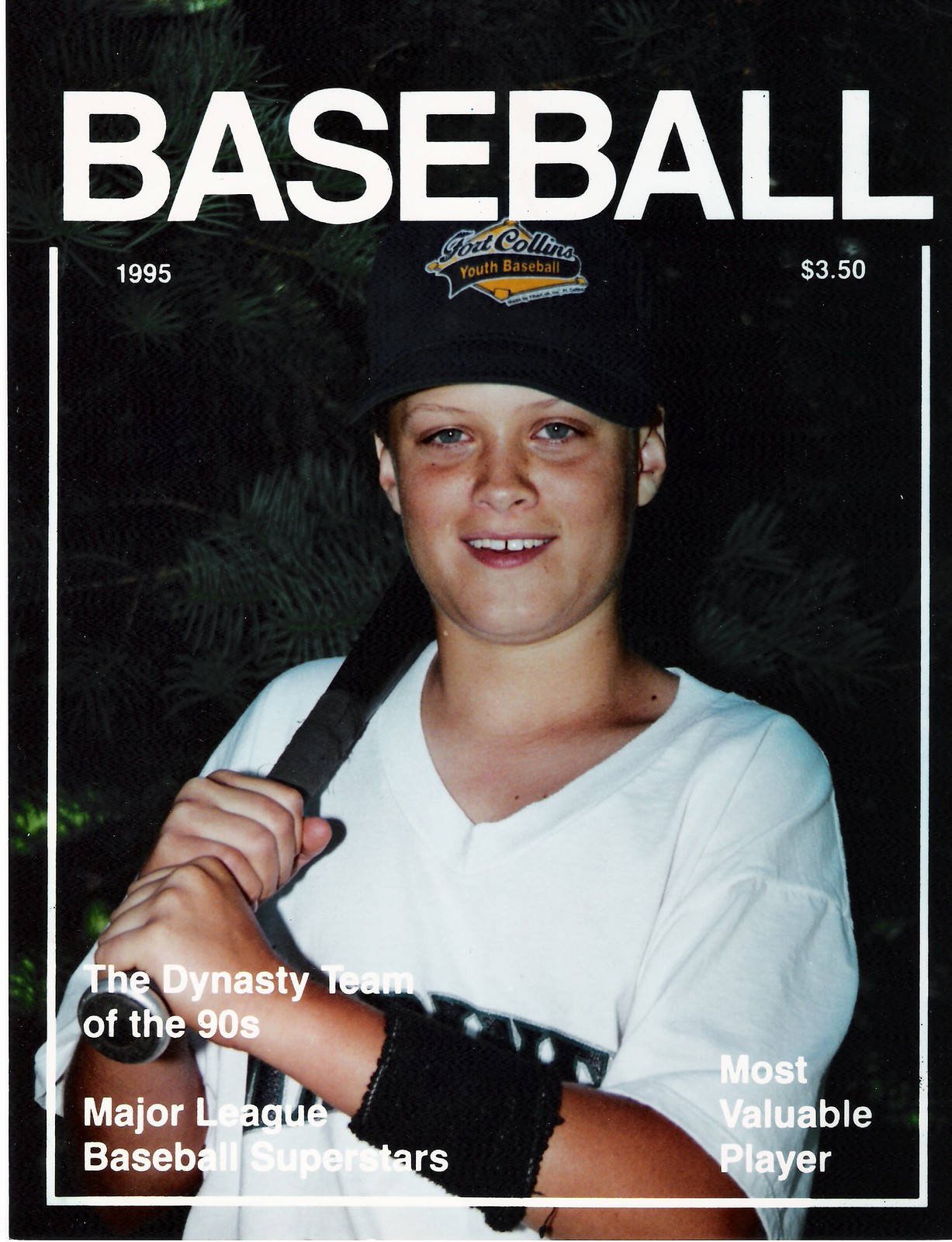The cover of this baseball magazine features a young boy of about 12 years old, set against a black background. At the very top, in large white letters, it prominently displays the word "Baseball," beneath which it says "1995" to the left, and "$3.50" to the right. The cover image is a portrait of the boy, with a slight smile revealing his top teeth and a small gap. He has blue eyes and is wearing a black baseball cap inscribed with "Fort Collins Youth Baseball" and a white V-neck jersey, though the team logo on the front is obscured by his arm. The boy is gripping a black bat with both hands at the bottom, and holding it over his right shoulder. On his left forearm, he sports a black wristband. Behind him, there appears to be a green fern tree. In white letters near his hands, the text reads "The Dynasty Team of the 90s," followed by "Major League Baseball Superstars" and "Most Valuable Player" at the bottom right.